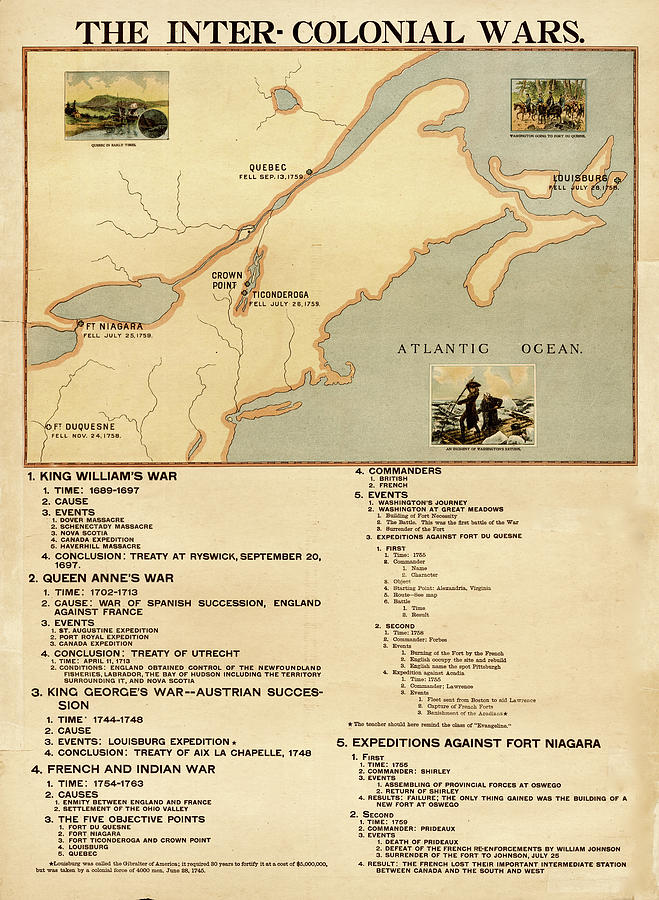This image displays a detailed historical map titled "The Intercolonial Wars," prominently indicated in bold black text at the top. The map encompasses a geographical representation with the Atlantic Ocean situated in the bottom right corner. Important locations such as Fort Niagara, Crown Point, and Quebec are highlighted, suggesting a focus on regions that may be part of Canada. Additionally, the map is interspersed with text boxes that outline significant historical conflicts, including King William's War, Queen Anne's War, and the French and Indian War. Each box provides comprehensive information such as the dates, causes, key events, and conclusions of these wars, offering a thorough historical context.